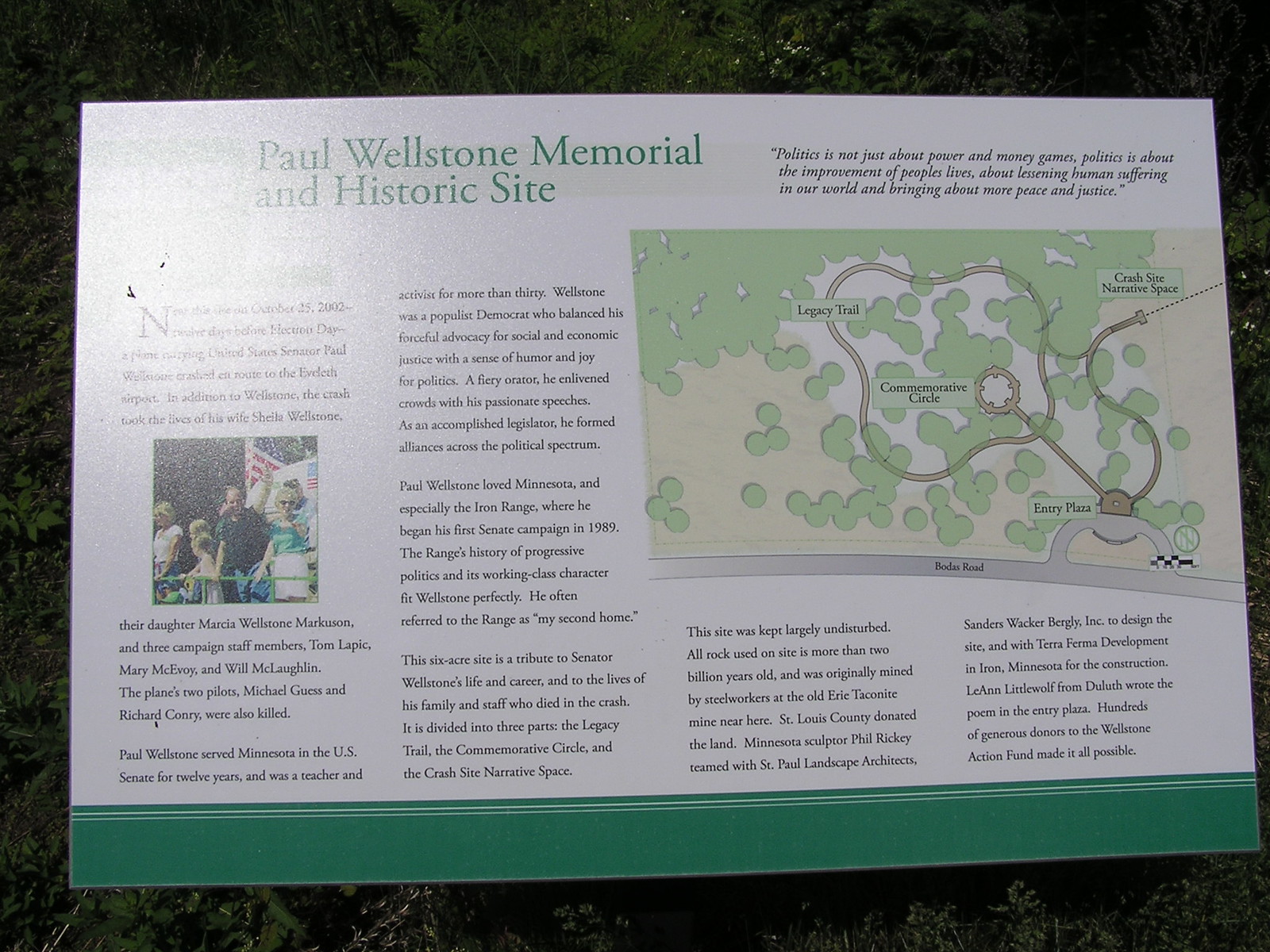This photograph captures a detailed outdoor sign for the Paul Wellstone Memorial and Historic Site. The sign is predominantly white, accented by a green stripe running along the bottom. At the top left, the sign states "Paul Wellstone Memorial and Historic Site" in green text. Adjacent to this, on the right side, is an inspiring quote: "Politics is not just about power and money games. Politics is about the improvement of people's lives, about lessening human suffering in our world, and bringing about more peace and justice."

Beneath the quote, there is a small map guide featuring cartoon-like trees and a circular trail. This map labels significant locations such as the Legacy Trail, Commemorative Circle, Entry Plaza, and Crash Site Narrative Space. On the left side of the sign, there is a photograph of a few people standing in front of a flag, although the image is too small to make out clearly.

The sign is set against a backdrop of trees or bushes, indicating it is taken outside during the day, as evidenced by the natural lighting that makes all the details visible.